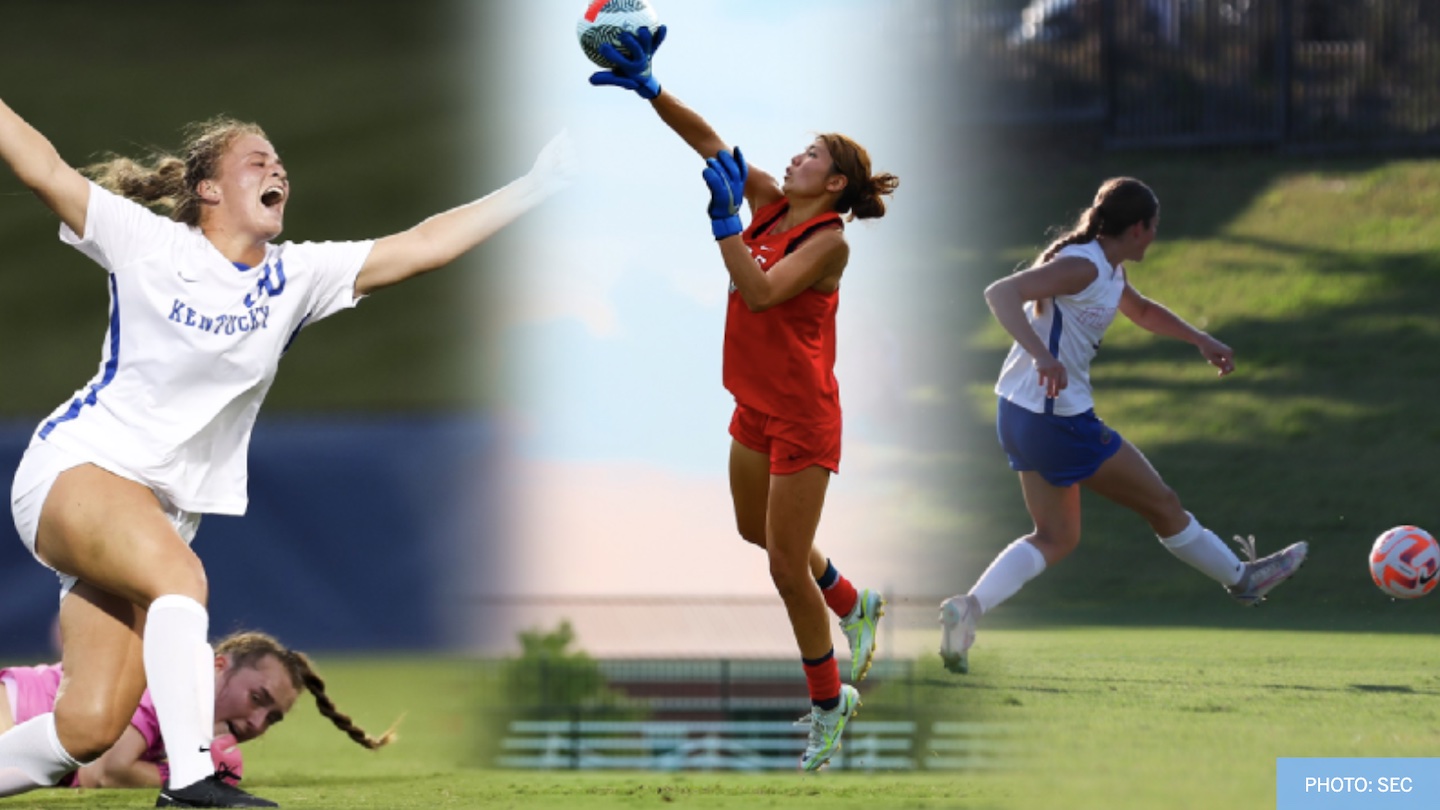This composite image showcases four distinct female soccer players engaged in various dynamic actions. The far-left panel features a blonde player enthusiastically celebrating, her arms raised and mouth open in a victorious yell. Donning a white Kentucky jersey with blue lettering, white shorts, white soccer socks, and black cleats, she stands over another player in a pink jersey sprawled on the green grass beneath her, suggesting a moment of triumph over an opponent.

The middle panel centers on an Asian-looking player dressed in a vivid red volleyball uniform, distinct from the soccer attire surrounding her. This player appears to be leaping or poised to hit a volleyball, her right palm up with a white, blue, and red volleyball resting on it, and her blue-gloved left hand extended. She's surrounded by a backdrop of blurred empty stands and white space, highlighting her airborne moment.

On the far right, another soccer engagement unfolds with a player kicking a white soccer ball adorned with orange and purple stripes. She sports a white jersey featuring a blue stripe down the side, blue shorts, white knee-high socks over her shin guards, and white and gray cleats. Her dark hair is pulled back in a ponytail as she executes her kick, her posture indicating mid-action intensity on a field of green grass.

Additional details such as the mention of “SEC” in white print on a blue rectangle in the bottom corner subtly anchor the image, emphasizing a scenario within collegiate athletics.